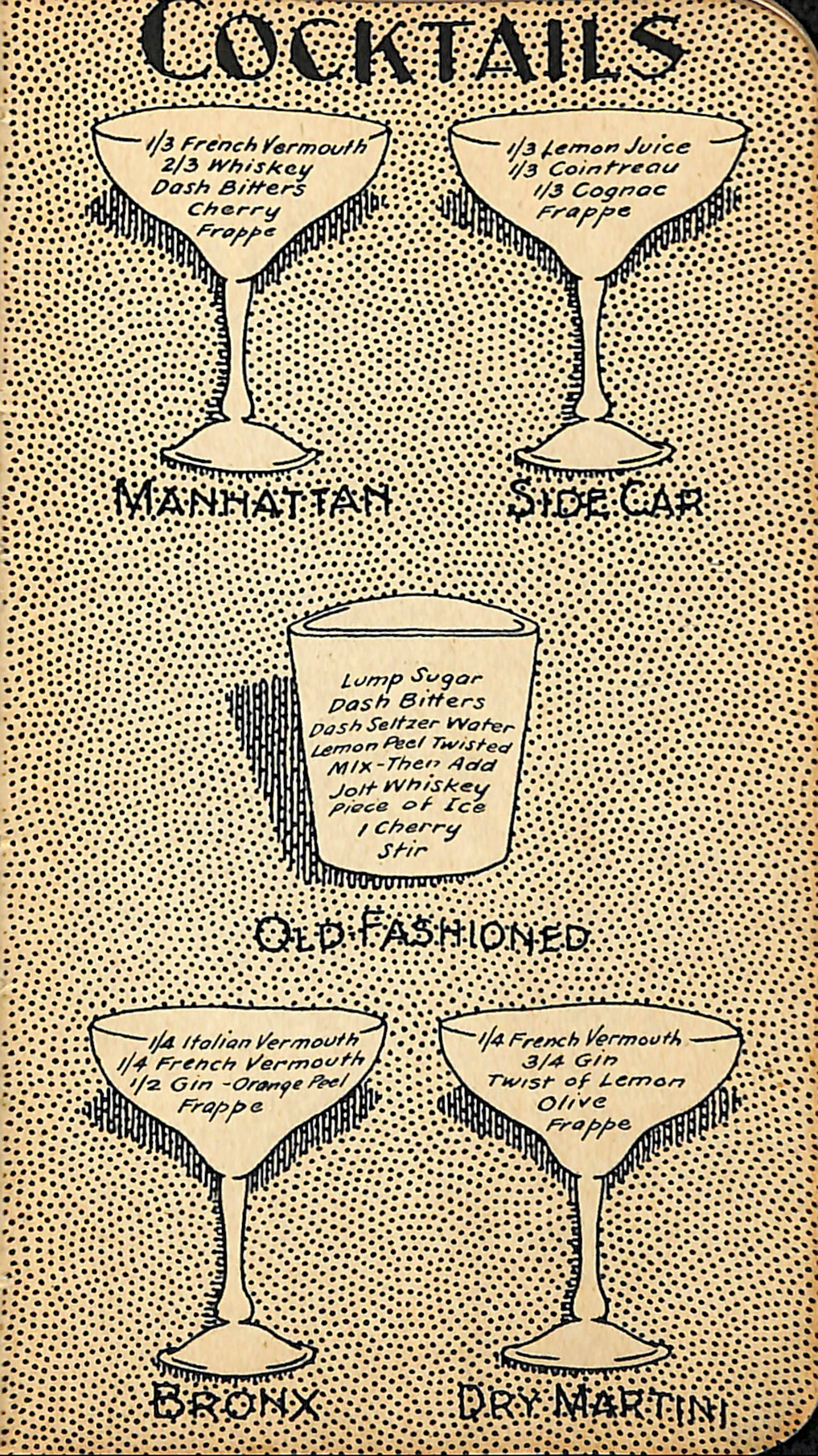The image is a detailed poster showcasing five cocktail recipes against an aged beige paper backdrop with a pattern of small, closely-spaced black dots, creating an optical illusion effect that can strain the eyes. The top of the vertical rectangular poster features the title "Cocktails" in bold black letters. Directly beneath the title, there are two martini glasses side by side, labeled "Manhattan" and "Sidecar," respectively. The Manhattan recipe calls for one-third French vermouth, two-thirds whiskey, a dash of bitters, a cherry, and frappé. The Sidecar recipe includes one-third lemon juice, one-third Cointreau, one-third cognac, and frappé. Below these is a section with a single old-fashioned glass, detailing the ingredients for an "Old-Fashioned": lump sugar, a dash of bitters, a dash of seltzer water, a twisted lemon peel, mixed with a jolt of whiskey, a piece of ice, and one cherry, stirred. At the bottom of the poster, there are two more martini glasses. The left glass is labeled "Bronx," with its recipe calling for one-fourth Italian vermouth, one-fourth French vermouth, one-half gin, an orange peel, and frappé. The right glass is labeled "Dry Martini," and its recipe includes one-fourth French vermouth, three-fourths gin, a twist of lemon, an olive, and frappé. The image is vividly lit, presenting each cocktail recipe clearly.